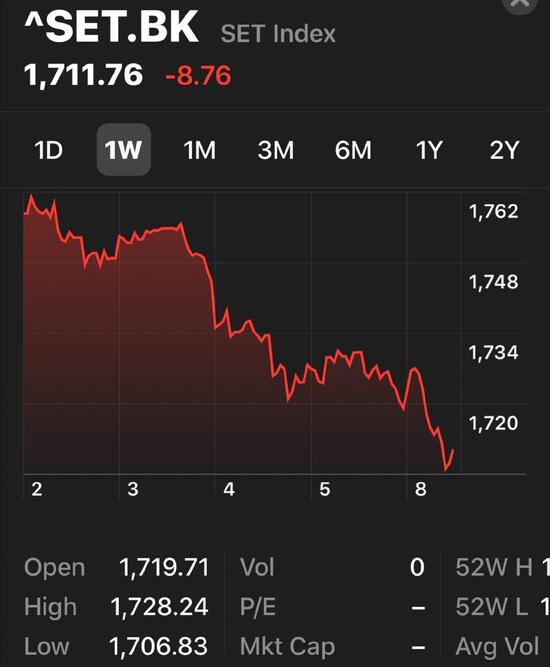The image features a primarily black background displaying key financial information. At the top, it reads "SET.BK Set Index" with the current index value prominently shown as "1711.76," representing a decline of "8.76 points." Below this, various time frames are indicated: "one day," "one week," "one month," "three months," "six months," "one year," and "two years."

A graph occupies the lower portion of the image, with horizontal axis values ranging from "2" on the left to "8" on the right, and vertical axis values spanning from "1762" at the top to "1720" at the bottom. The plotted curve starts high on the left side of the graph and slopes downward to a lower value on the right side, reflecting a decreasing trend.

Additional financial metrics are displayed beneath the graph: the opening value is "1719.71," the highest value reached is "1728.24," and the lowest value is "1706.83." Other indicators include "VOL 0," "P/E -", and "MKT cap -", along with "52 WH -," though specific figures for these metrics are not provided.